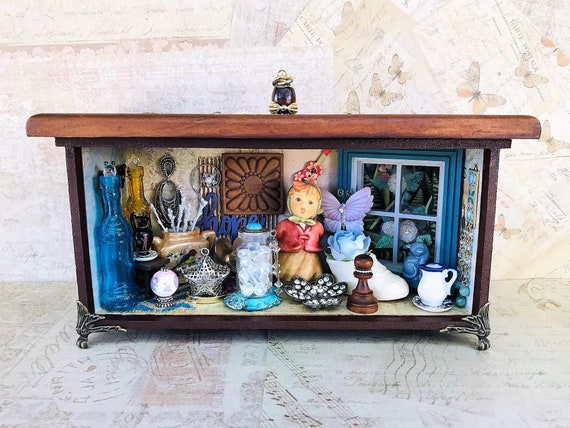This is a color photograph of an eclectic and cozy shadow box designed to display small collectibles. The shadow box is crafted from dark red wood, featuring ornate pewter or silver-covered metal legs. The background is creatively adorned with decoupage, depicting faux letters, stamps, and butterfly images, enhancing its vintage charm. 

Inside the box, you'll find a variety of miniature antiques and trinkets meticulously arranged. On the left, there's a blue bottle, paired with a similar amber one, both possibly filled with marbles. A small, intricately painted Kewpie doll stands near a white shoe with a blue flower protruding from it. Among the collectibles is a tiny teapot, various small potteries containing dried flowers, a purple butterfly, a miniature silver star ornament, a wooden coaster, and a pawn chess piece made of the same wood as the display itself. 

Displayed alongside these items are a small teacup, a doll, a purple ball on a stand, and a little jug with plant matter coming out. Notably, there's a decorative blue and white window with fake plants behind it, adding depth to the background. Strings and ribbons hang on the wall, further enhancing the intricate and detailed assembly of this shadow box.